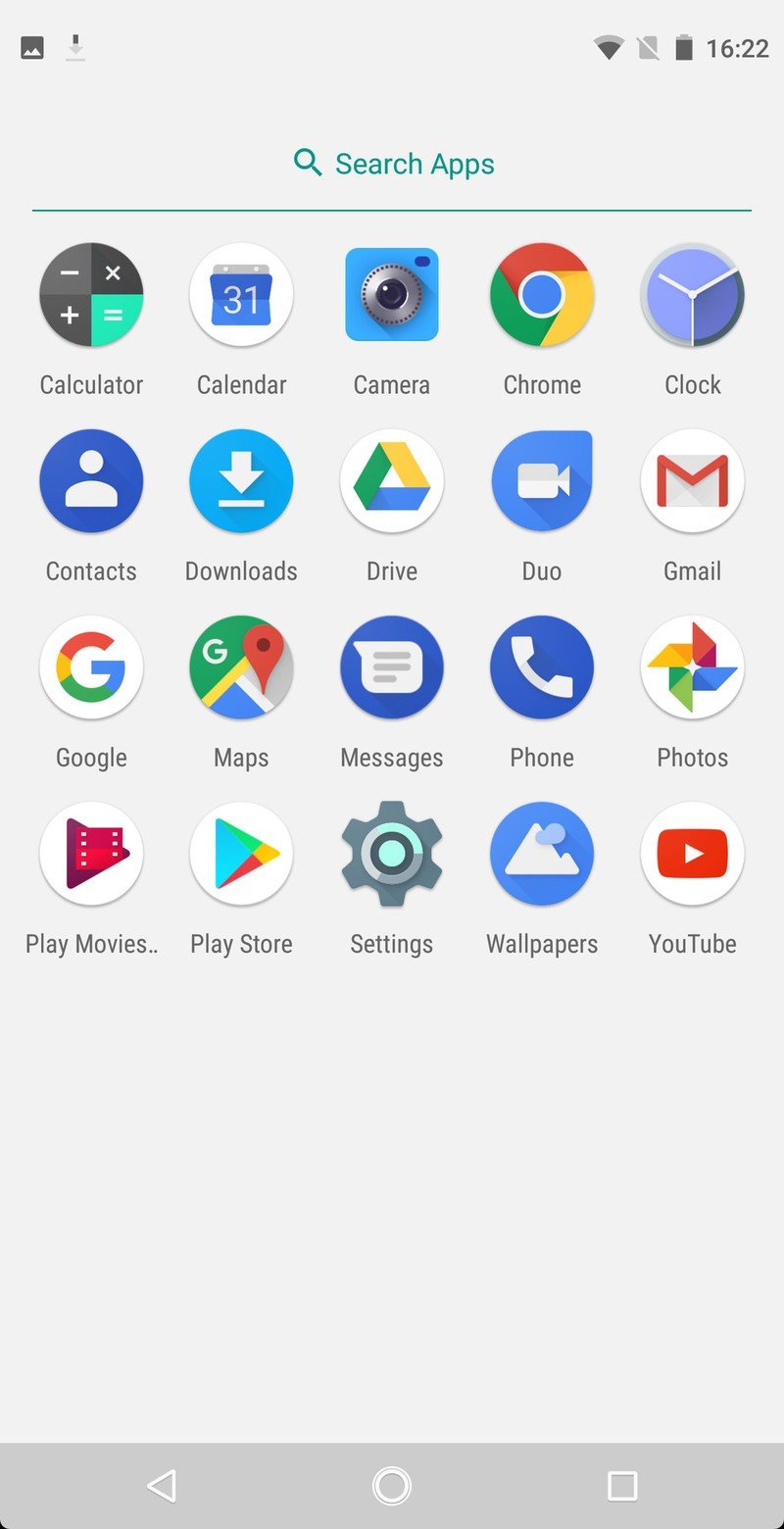The image showcases the app drawer of an Android phone featuring a light grey background. The drawer contains an array of predominantly pre-installed apps neatly arranged within circular icons, with notable inclusions being Calculator, Calendar, Camera, Chrome, Clock, Contacts, Downloads, Drive, Duo, Gmail, Google, Maps, Messages, Phone, Photos, Play Movies, Play Store, Settings, and YouTube. Each app icon maintains a uniform circular boundary, except for Duo, which adopts a unique teardrop shape, and the Camera app, exhibiting a slightly square outline. At the top of the drawer, there's a gear icon symbolizing settings, a search bar for easy navigation, and intriguingly, a Wallpapers app, which might suggest some degree of customization. The organized and minimal setup implies that the phone may have been recently booted up for the first time or the user prefers to keep their app selection streamlined to essential functionalities.